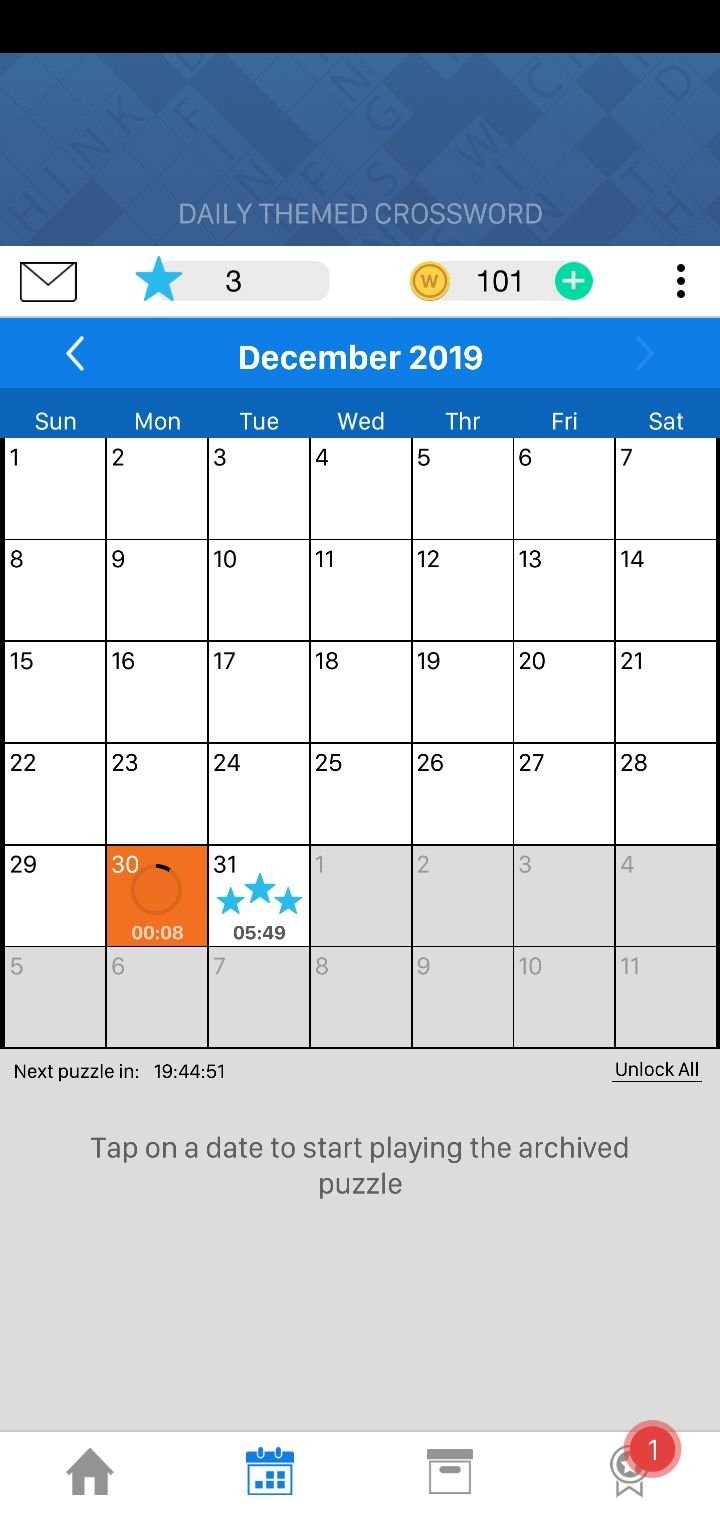Archived Calendar of Daily-Themed Crossword Puzzles:

At the very top of the image is a thin black rectangle running horizontally across the page. Directly beneath it is a darker blue rectangle with light blue text centered at the bottom reading "Daily Themed Crossword." Below this, from left to right, are an envelope icon, followed by a blue star icon, and the number "3." Further right, there is a yellow circle with a brown "W" in the center, followed by the number "101," and a gray circle with a plus sign inside it. To the farthest right are three vertical black dots.

Beneath this row is another blue rectangle with white text. From left to right, it displays a white directional arrow pointing to the left and the text "December 2019" in the center. Below this, there is the calendar for December 2019, which spans from Sunday to Saturday for the entire month. The date "Monday, December 30th" is highlighted in orange with a central circle displaying "00:08." December 31st features three blue stars and the time "05:49."

Below the calendar, the text reads "Next Puzzle in 1944:51," and to the right, there is the option "Unlock All." At the bottom of the image, there is a prompt that says, "Tap on a date to start playing the archived puzzle."